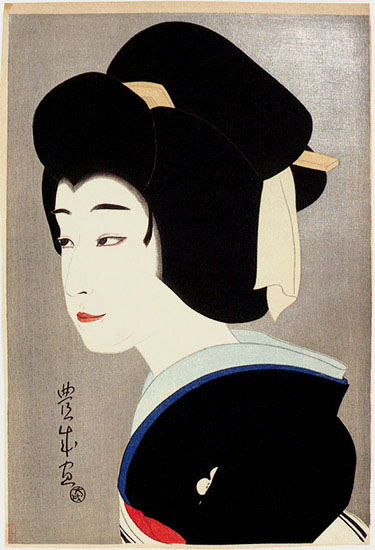This is a painting or a print of a traditional Japanese portrait of a woman in profile, most likely a geisha. The woman, with her fair white face and neck, is depicted looking to the left. Her dark eyebrows and eyes contrast with her red lips, creating a striking facial expression. Her black hair is styled into a large bun with a chopstick or hairbrush inserted, adorned with a white headdress or headscarf that drapes from the back of her head. She wears a black kimono with a blue collar, a touch of red near the belt area, and a white flower or accent on the shoulder. The background is primarily gray or light brown, featuring a series of Japanese characters towards the bottom left corner, adding to the cultural authenticity of the piece. The artwork, likely created with watercolor techniques, beautifully blends traditional elements with intricate details to capture the essence of Japanese elegance. The woman appears to be smiling slightly, enhancing the portrait's serene and graceful ambiance.